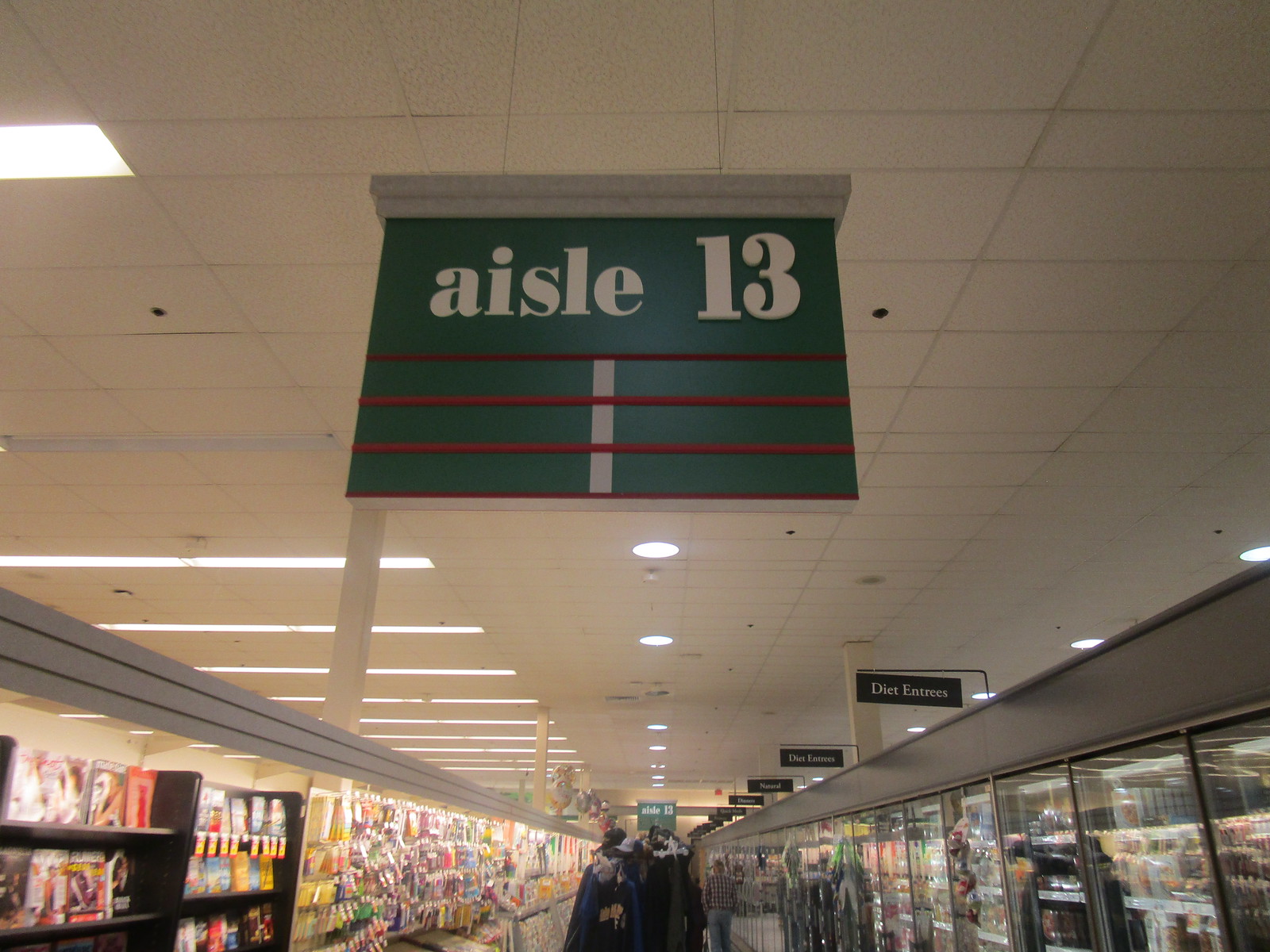This detailed photograph captures an aisle in a supermarket, specifically a refrigerated and frozen food section clearly marked as "Aisle 13" with white lettering on green signs accented by red stripes at both the front and back of the aisle. The ceiling features a white and gray speckled drop ceiling design, complemented by fluorescent lighting on the left side and circular cutout lights running along the middle. On the right side of the aisle, gray-topped coolers with glass doors store various food items, with hanging signs above indicating sections such as "diet entrees." On the left, there are hanging displays and packages of cheese, yogurt, and prepared meals. In the center aisle, clothing racks and office supplies are interspersed among magazine displays. A man in a white and dark checked shirt with blue jeans walks away from the camera towards the back of the aisle. Additional signage, though partially unreadable, suggests the presence of natural food items further down the aisle.